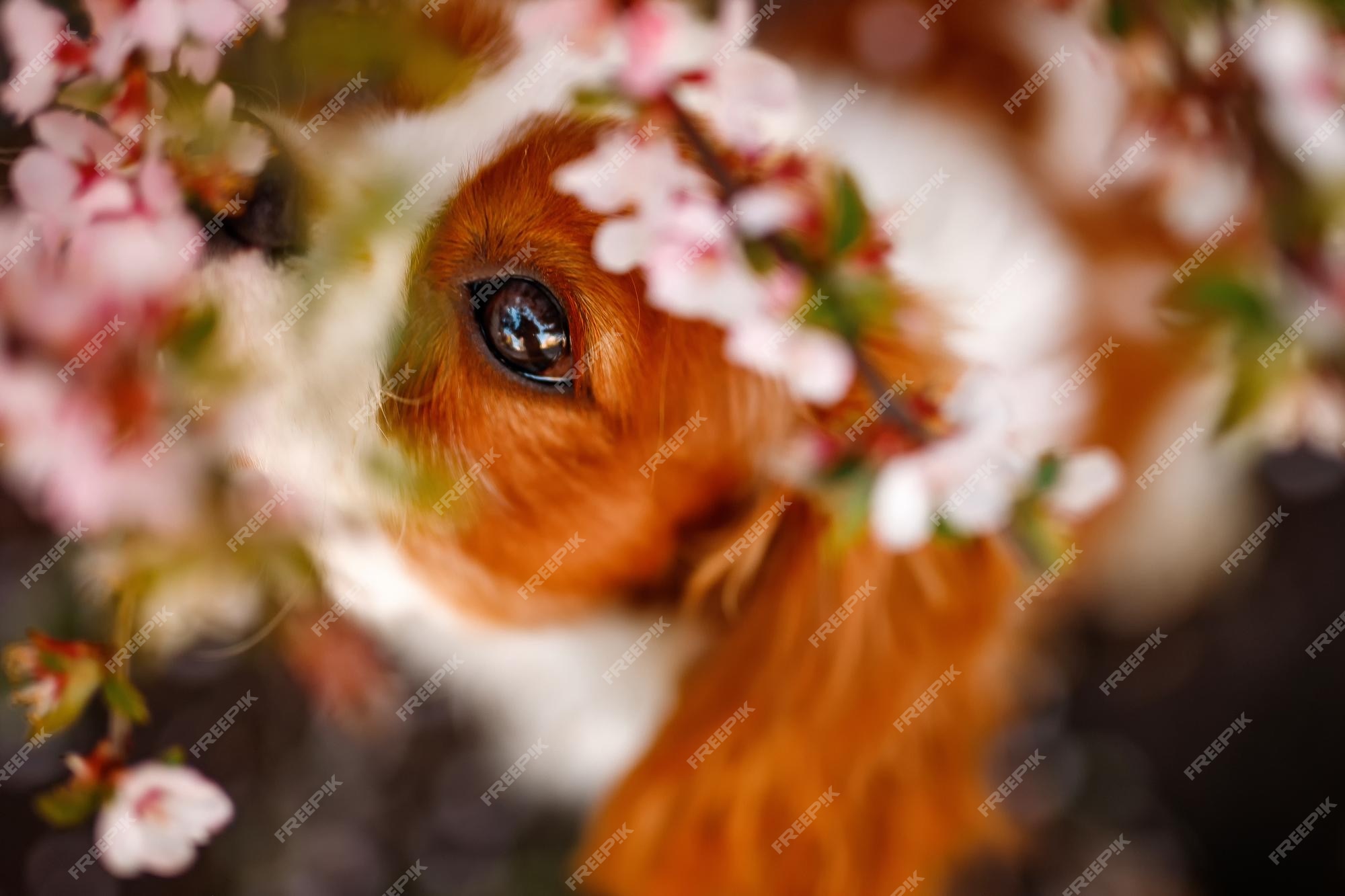This nature image, embedded with a repetitive diagonal white watermark reading "free pic," features a contrasting composition of blurred and sharply focused elements. The blurry backdrop showcases a mixture of green leaves, white flowers, and predominantly pink blooms, likely cherry blossoms, clustered around the edges. Amidst this floral setting, the lone clearly focused elements are a portion of an animal's face and its keen eye. This eye, framed by light brown and white fur, likely belongs to a small dog, possibly a cocker spaniel or a Cavalier King Charles Spaniel. The dog's wide eye suggests an intense curiosity as it sniffs among the blossoms, with its floppy ears partially visible despite the overall blurriness of the photo. Despite the imperfections, the sharp focus on the eye and the surrounding fur conveys a sense of intrigue and engagement with the natural surroundings.